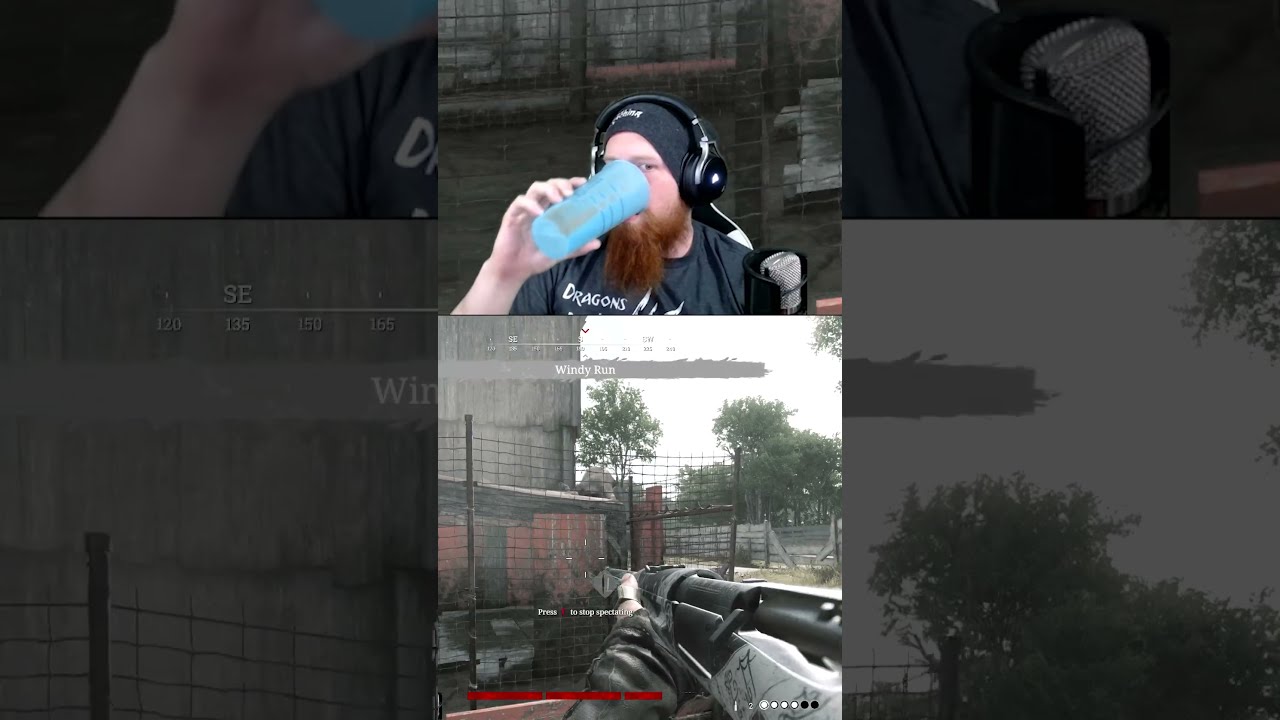The image is a collage of six photographs, displaying close-ups and medium shots centered around two primary images. The central top image features a bearded white male, with a reddish-brown beard and a black stocking cap. He's wearing over-the-ear headphones and drinking from a blue plastic cup. He is also in front of a microphone, suggesting he might be a radio jockey or a gamer. The man is wearing a black t-shirt with "Dragons" printed on it. Behind him, there are cassettes and a steel fence, typical of a cluttered set-up.

Directly beneath this image is another key photograph depicting a scene from a first-person shooter game. This scene shows an outdoor setting in a village or town with a slightly decrepit atmosphere, evidenced by a wooden fence and a concrete building in disrepair. The game screen includes the text "Windy Run" at the top. At the bottom of this game image, a hand holds an automatic rifle towards the building, with a visible red health bar in the corner. Trees can be seen in the background.

The four surrounding panels are close-ups of these two central images: the upper left shows the man's wrist and part of his shirt and blue cup; the upper right focuses on the microphone; the lower left displays a close-up of the building; and the lower right captures the trees behind the building. The peripheral close-ups are slightly blurred, emphasizing the central images.